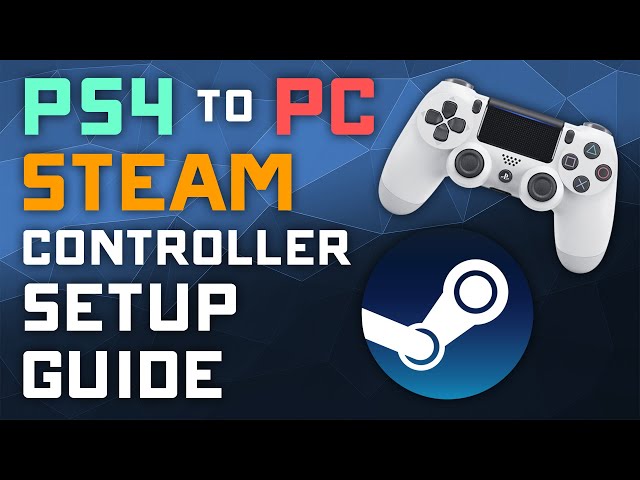The digital art image appears to be a detailed thumbnail for a YouTube video tutorial on setting up a PlayStation 4 controller for use with a PC on the Steam platform. The background features deep blue hues with geometric shapes creating a textured appearance, including rhombuses and triangles. Overlaying the background are two long rectangular black bands, one at the top and one at the bottom, adding contrast and framing the design. The central and prominent text, "PS4 to PC Steam Controller Setup Guide," is written with varying colors: 'PS4' in light green, 'to' in white, 'PC' in red, 'Steam' in orange, and 'Controller Setup Guide' in white. To the top right of the image, there is a white PlayStation 4 controller with grey buttons. The arrangement and color choices highlight the step-by-step guide's intent, making it visually appealing and informative for viewers looking to set up their controllers for PC gaming on Steam.